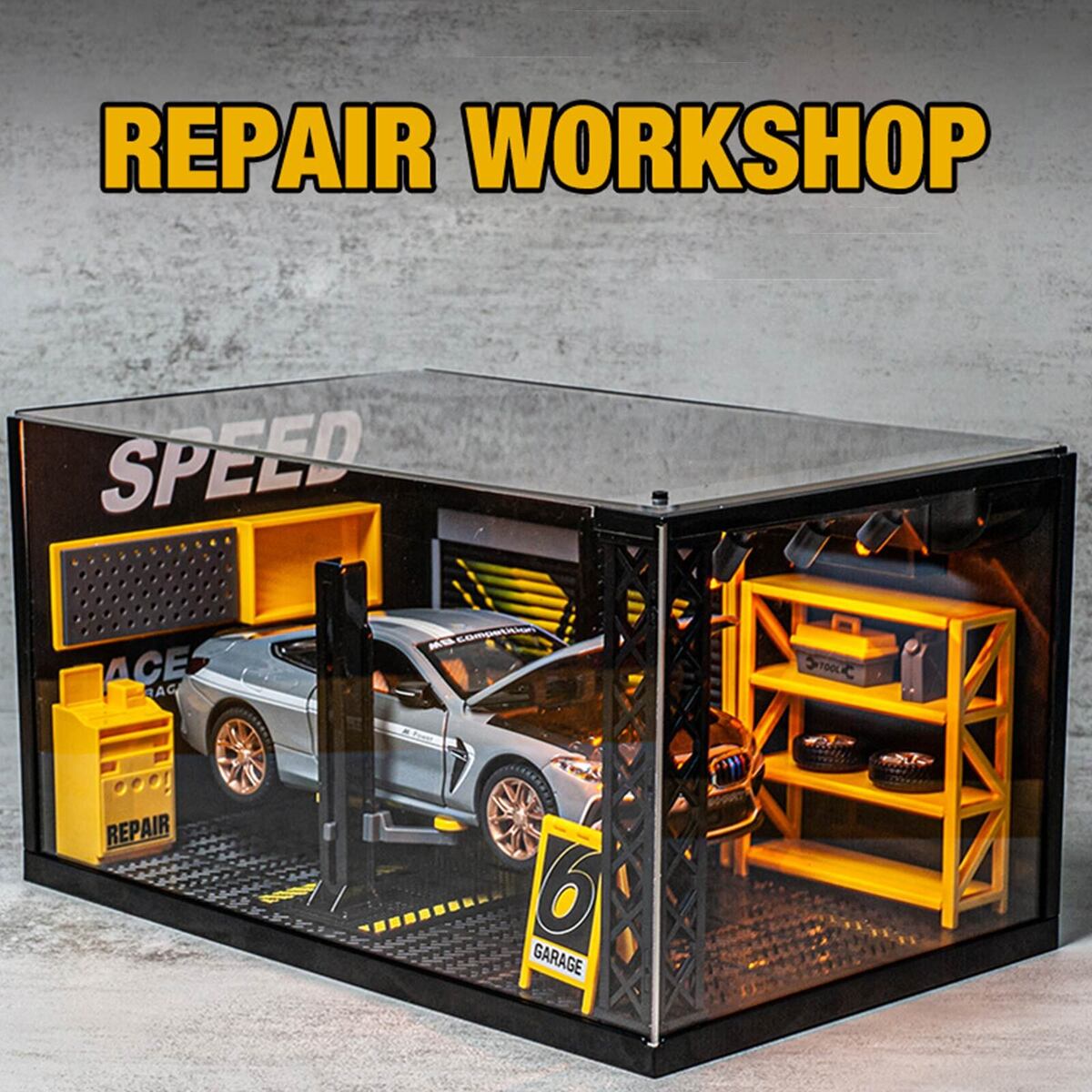This highly detailed, square-format color photograph depicts a 3D model car display encased within a clear, rectangular plexiglass box. The overall dimensions of the box are approximately five inches by five inches. The setting inside the box portrays a detailed garage car workshop scene.

Inside the box, a blue sedan sits prominently, lifted on a black garage jack in the center. The car has its hood open, revealing the detailed interior. Beneath the car, the floor features a grid pattern and rubber matting, adding realism to the display. 

To the left of the car, a yellow workbench stands, with the word “REPAIR” printed in black letters across the bottom. Above the car and in the back portion of the box, a multi-shelf unit with yellow shelving contains a couple of tires and various tools. On the back left wall, the word “SPEED” is boldly printed in large white italic letters.

The outer background of the image is gray with darker worn areas, and the top features a large golden yellow title with a black outline that reads “REPAIR WORKSHOP.” Towards the front right corner of the display, where the two sides meet, a small stand-up sign features a black background with the word “GARAGE” hanging on a white strip.

The overall style is photographic representationalism realism, capturing the intricate details and essence of a small-scale car workshop with impressive clarity.